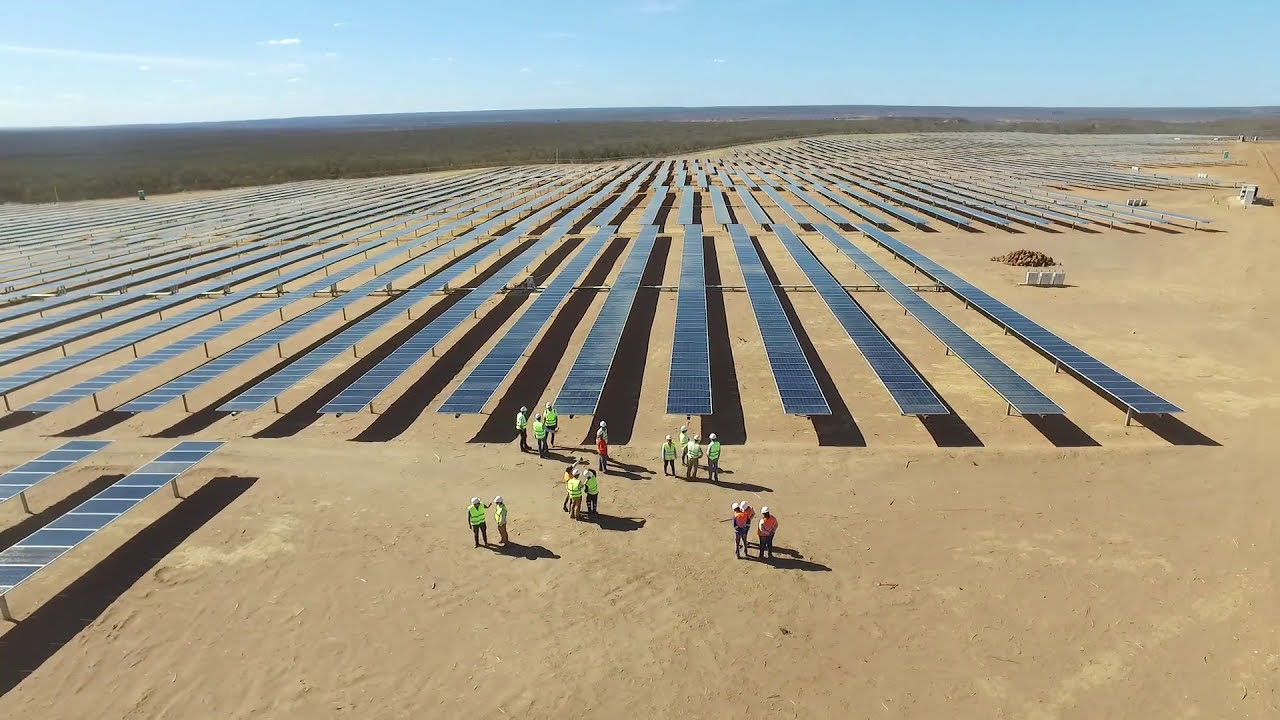This photograph, taken from an overhead perspective on a cloudless day, captures an expansive solar farm sprawling across a sandy, desert landscape. Dominating the upper two-thirds of the image are multiple horizontal rows—at least 12—of long, rectangular solar panels stretching towards the horizon, creating a striking pattern against the flat terrain. Each panel casts a distinctive shadow onto the sand, enhancing the geometric beauty of this renewable energy installation.

In the lower third of the image, five distinct groupings of approximately 15 workmen collectively stand in bright neon yellow and orange vests, complemented by white safety helmets. These individuals appear to be engaged in discussion, their formation suggesting organizational deliberation rather than active labor. The sandy ground below them enhances the industrial feel, devoid of greenery, buildings, or significant vehicles, save for two small vehicles faintly visible to the right.

Overall, the image presents a stark, clean juxtaposition of human activity against the pristine solar array under an unblemished azure sky, visually elucidating the magnitude and collaborative effort involved in harnessing solar energy in such a barren yet technologically advanced setting.